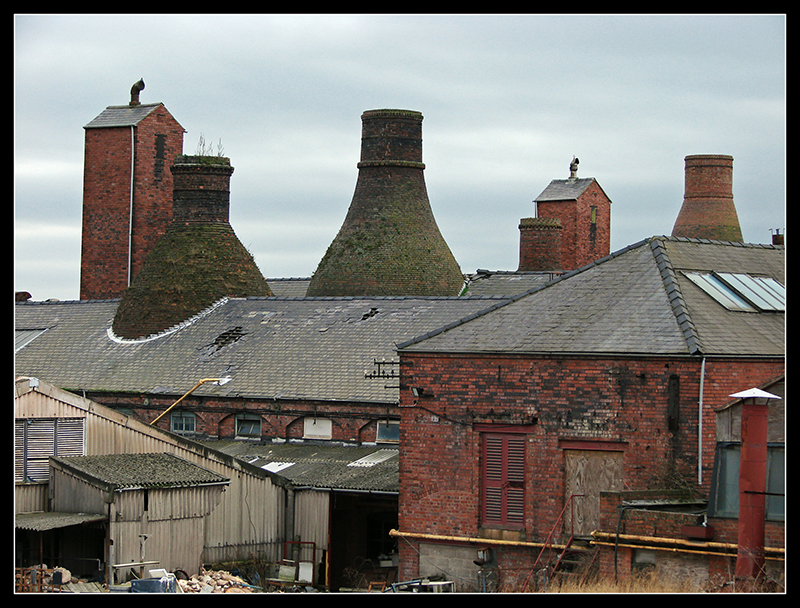The image depicts a collection of old, weathered brick buildings, possibly part of an abandoned factory or recycling facility. The building closest to the front is made of deteriorating red brick with dark, moldy spots and has no visible windows on its front-facing side. A red, slatted door and a boarded-up area—perhaps once a window or door—are present, along with a staircase descending from the boarded section. The roof is tiled with what appears to be a small window looking out from its top. Surrounding this structure are more brick buildings of various shapes and sizes, some featuring holes in their roofs and unique bottle-like air vents covered in green mossy plants. In the background, another structure is described as having a black roof, with red bricks covered in mold, alongside a silver building cluttered with debris such as paper and plastic bottles.